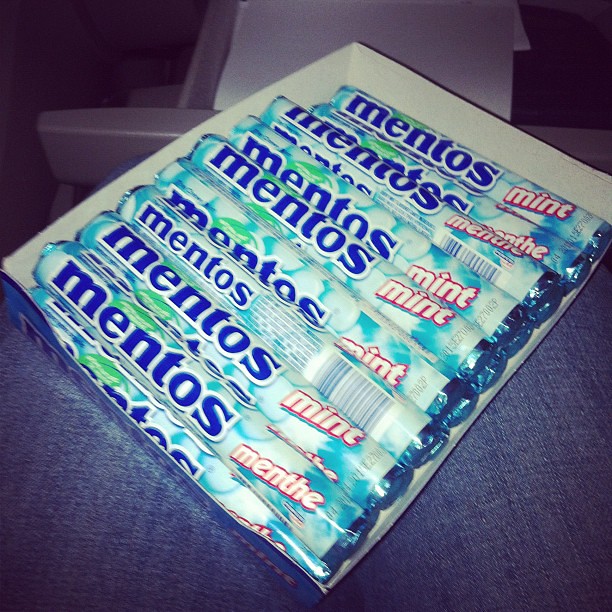This photograph features a close-up of at least ten rolls of Mentos mints, neatly organized in two rows within an open display box. The box, featuring a white interior and a blue exterior, is tilted diagonally with the top facing toward the top right corner of the image. It appears to be resting on a person’s knees, which are clad in blue denim jeans. The scene is illuminated by a flash, resulting in a slightly blurry effect. Dominating the background is a gray plastic chair, partially visible beneath the box. A purple filter casts a hue over the entire image, darkening the corners and highlighting the vivid colors of the Mentos packaging. The rolls, adorned with the word "Mentos" in dark blue, feature a light blue to green gradient with red and white text on the right side indicating "Mint." The packaging also includes shadowy imagery of the mint, with subtle green accents scattered throughout, adding to the detailed presentation of this everyday product.